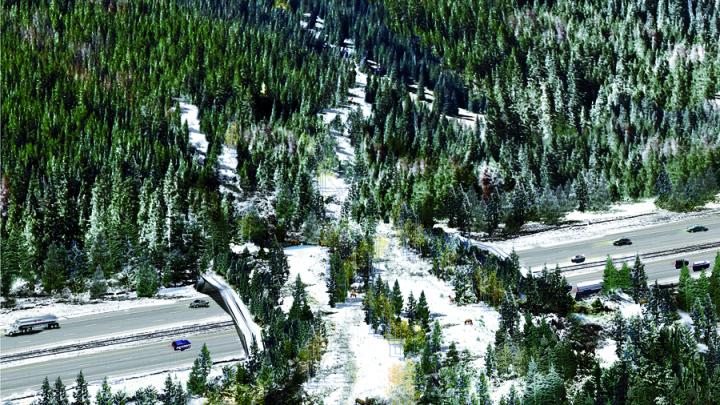The painting captures a snowy, outdoor scene of a highway stretching diagonally from the lower left to the middle right of the image. The highway features vehicles moving in both directions and is flanked by a snowy landscape abundant with pine trees. The trees, displaying varying shades of light and dark green with touches of white snow, are present both in the foreground and background, creating a dense forest that frames the scene. Above the highway, a snow-covered bridge, also lined with pine trees, spans the expanse, giving an impression of the forest extending over the road. Snow blankets the entire landscape, accentuating the wintery atmosphere. The intricate color details and the composition of the scene suggest it could be a highly detailed painting rather than a photograph.